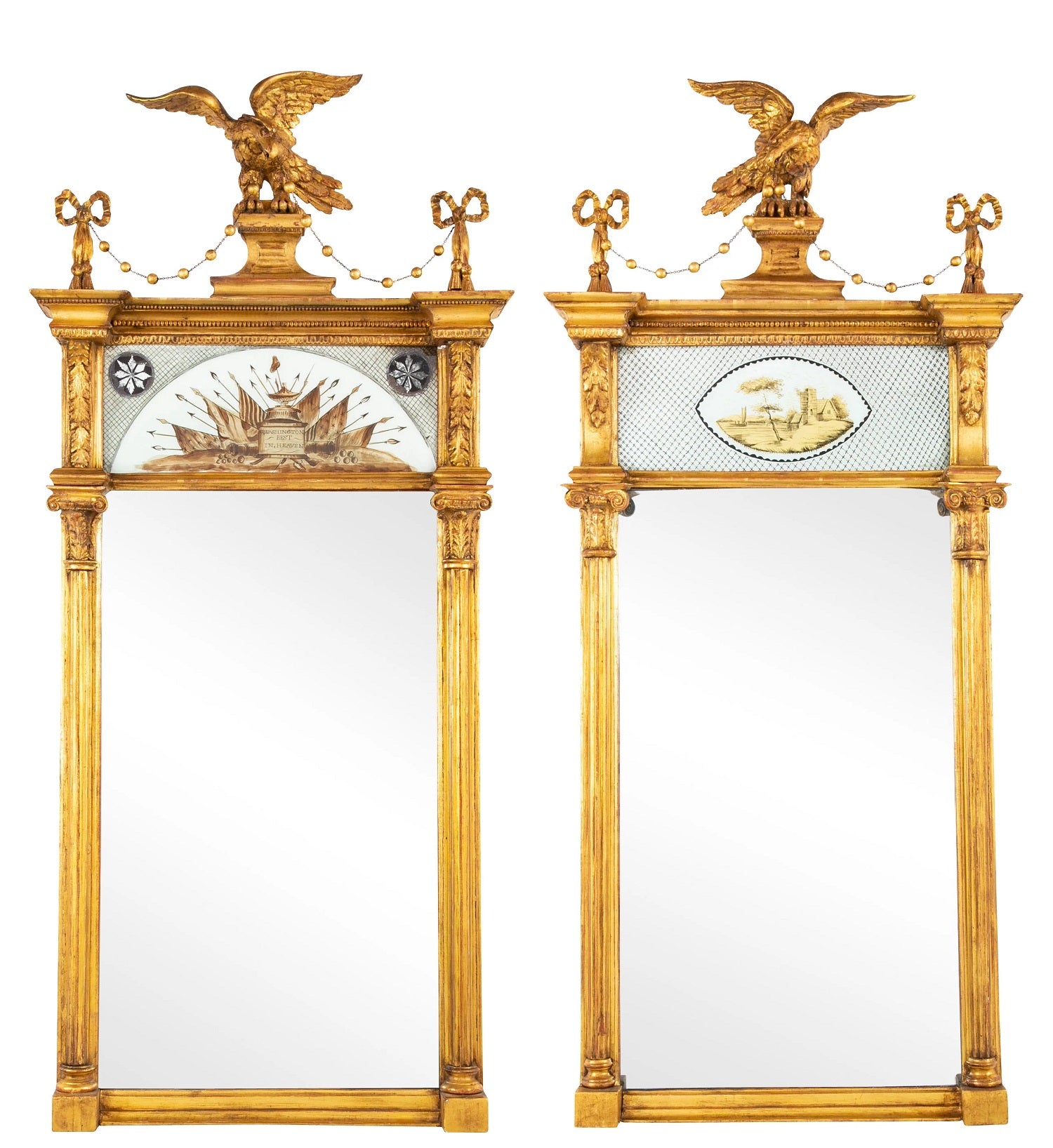The image features two ornate, rectangular wooden structures, each potentially serving as mirrors or windows, set against a white and gray backdrop. The wood is finished in an opulent gold color, showcasing intricate carvings and detailed designs. Both structures are framed by slender columns on the left and right, with a decorative base and an elaborately ornate top. At the pinnacle of each structure stands a majestic gold statue of an eagle, with wings spread, perched on a pedestal. These eagles are flanked by smaller animal figures on both sides.

Beneath the eagle on the left structure, there is an oval-shaped artwork, featuring two flowers in a circle surrounding an indiscernible structure with protruding elements. The eagle atop this structure faces forward, while the one on the right is turned around, revealing a cross pattern and a football-shaped design amidst various indistinct images dominated by white and yellow hues.

Connecting each statue to the main frame are metal, scissor-like ornaments imbedded into the wood, adorned with chains and beads. The sophisticated carvings extend across and down the sides, adding to the luxurious and detailed nature of the entire piece.